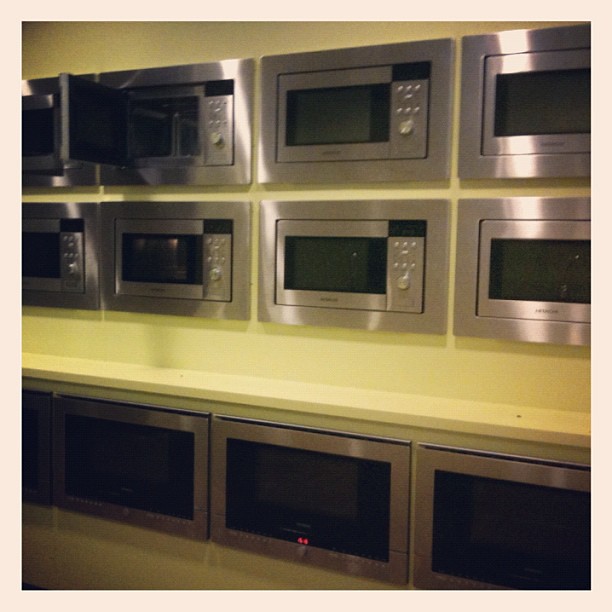The image shows a showroom display of kitchen appliances, specifically a series of wall-mounted, stainless steel microwaves and ovens. The arrangement consists of approximately 10 to 12 microwaves, each featuring several buttons, a turn knob, and some with doors open, set against a yellow matte wall with a beige border. Below the microwaves are larger oven doors, likely part of the same ensemble. These units, possibly including convection ovens, appear in two different levels with the controls located in the upper units. The lighting is a low fluorescent, making the image slightly grainy and out of focus, while a flash reflection creates a glare on the stainless steel surfaces. Despite the photo's imperfect quality, the setting suggests a store specializing in kitchen appliances.